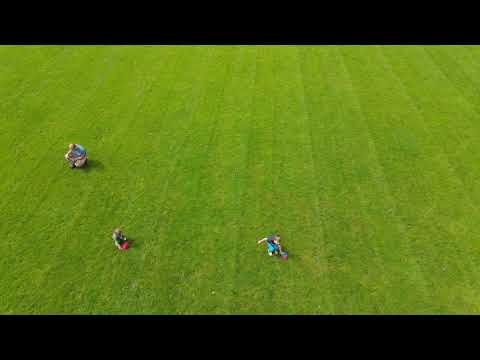This image, framed by black horizontal bars at the top and bottom, presents an overhead aerial view of a freshly mowed green grass field. The grass features defined vertical mowing lines adding texture to the scene. In the left third of the image, two people can be seen from above, standing on the grass. One person is situated slightly higher than the other. Both appear to be involved in an activity that suggests bending or crouching, potentially with a red and a purple item. In the bottom middle third of the image, a third individual, dressed in blue, is similarly engaged in the field. The image, likely captured by a drone, gives an impression of a garden or field where three people seem to be working, possibly gathering something into containers.